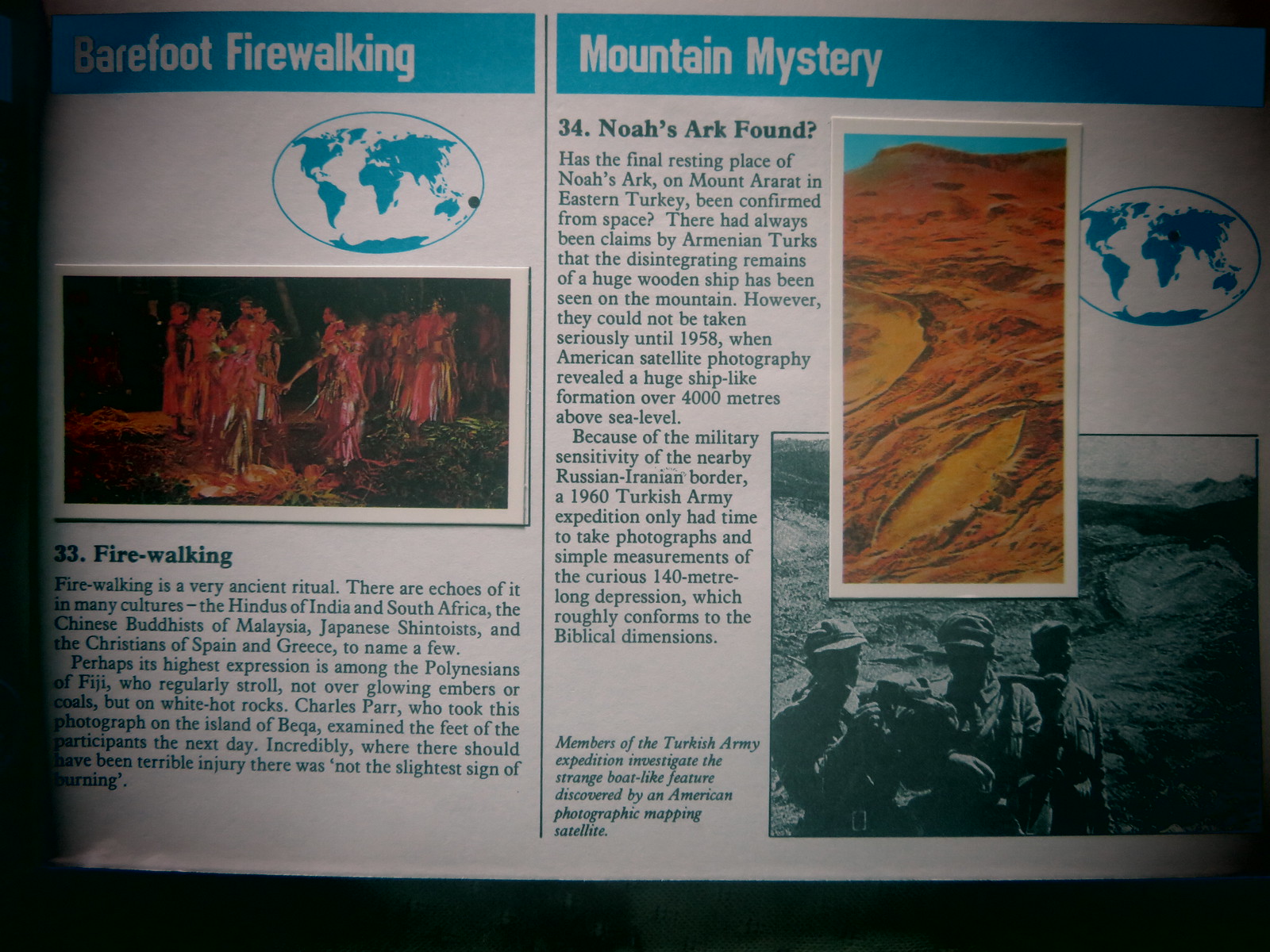This image appears to be an informational booklet or sign. On the left half, the title "Barefoot Walking" is displayed at the top next to an image of a globe with a marked location. A photograph beneath this title depicts individuals who are seemingly performing a fire-walking ritual. The text, labeled as "33. Firewalking," describes fire walking as an ancient ritual practiced by various cultures, including the Hindus of India and South America, the Chinese Buddhists of Malaysia, Japanese Shintoists, and Christians from Spain and Greece.

On the right half of the page, the section titled "Mountain Mystery" is introduced at the top, with "34. Noah's Ark Found?" immediately below it. Another globe indicates a different location pertaining to this topic. This section includes two photographs: one of a desert landscape and another in black and white showing members of a Turkish Army expedition examining peculiar boat-like features, which were discovered by an American photographic mapping satellite. The accompanying article provides more detailed information about this discovery and its historical significance.